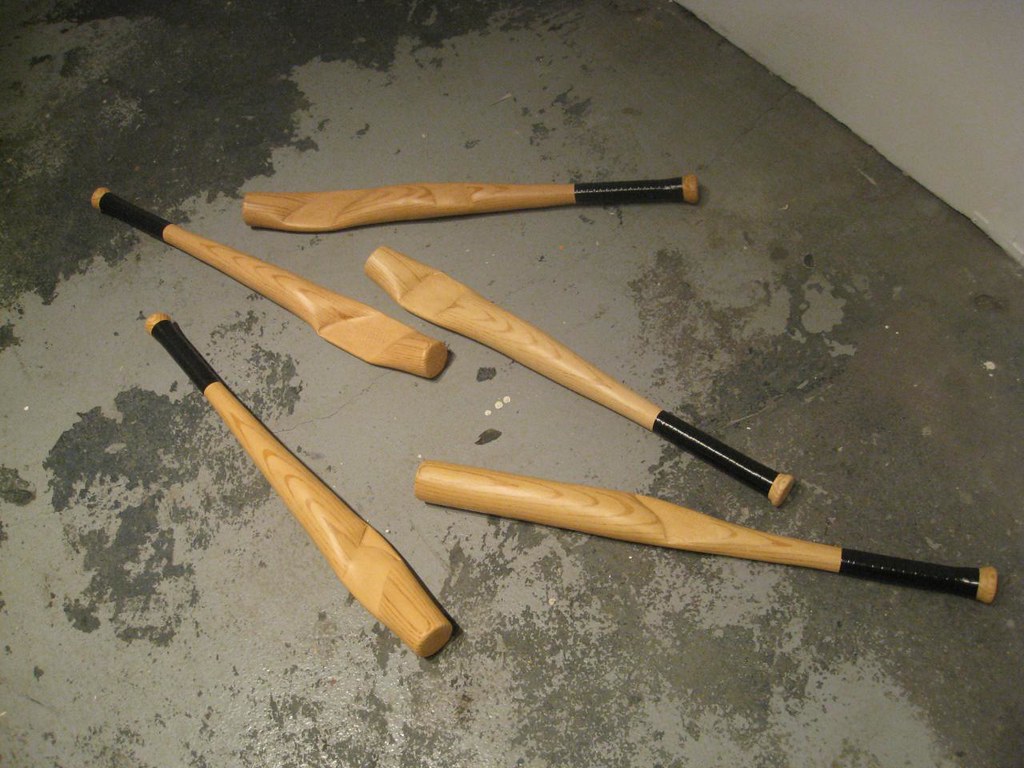This is an image of five beige baseball bats with black tape around their handles, laid out on a gray, wet concrete floor. Four of the bats are dented, with significant damage evident at their tops, causing them to lay flat against the ground. Despite being made of plastic, the bats are designed to mimic real wood, featuring striations that resemble a wooden grain. The backdrop of the image includes a tan wall that connects to the concrete floor, giving the impression that the scene is taking place in a garage or a basement. The colorful contrast between the beige bats and black tape provides a striking visual against the drab, concrete surface.